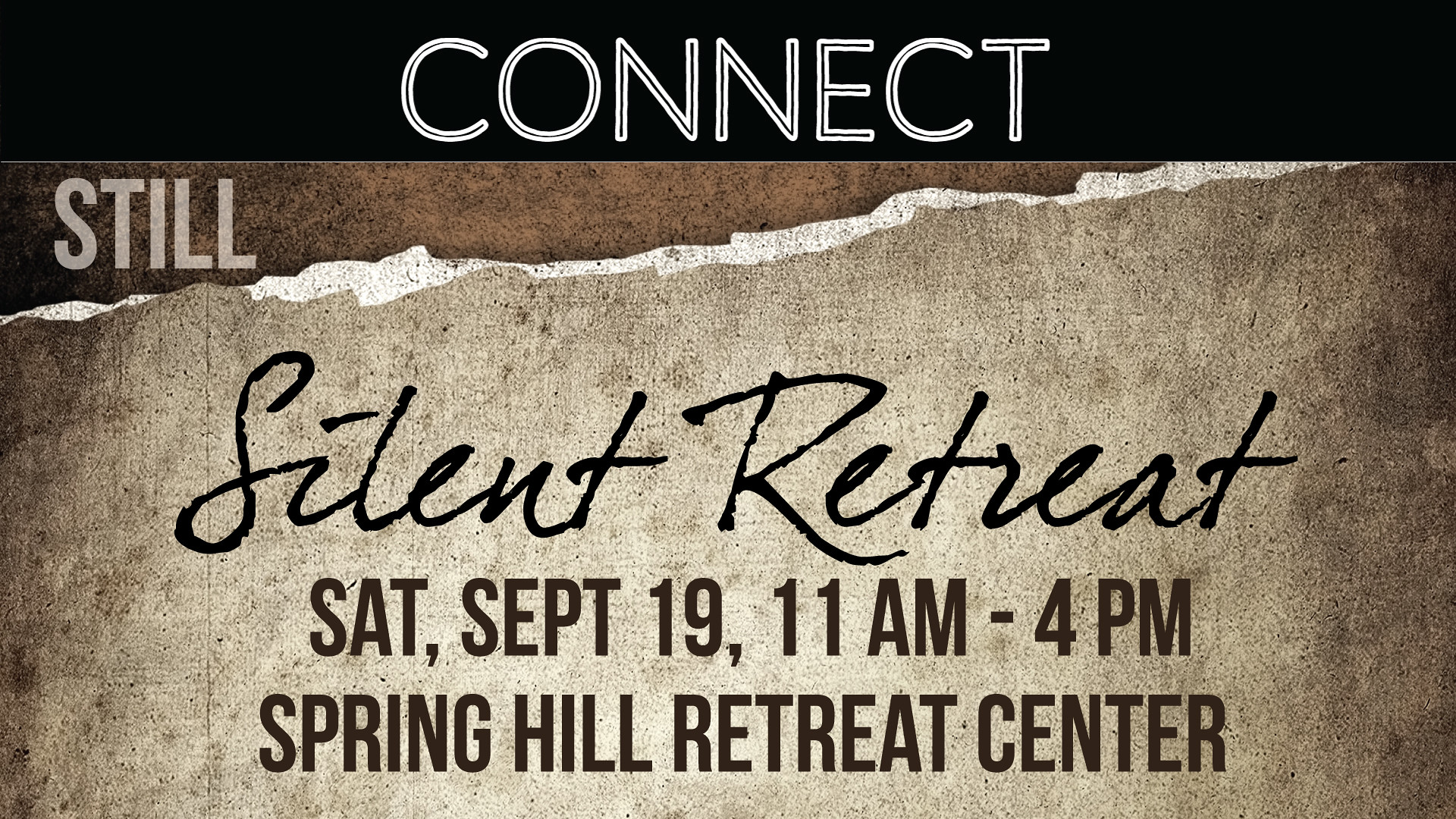The image is a digital flyer with a landscape orientation, styled to look like an aged, rustic piece of paper. At the very top of the image, a thin black bar spans approximately 20% of the width, featuring the word "CONNECT" in all caps, white text. Below this bar, the background consists of a mix of browns and grays, giving it a textured, vintage appearance. In the upper left corner in white text, the word "STILL" is displayed. Centrally located on the flyer, the words "SILENT RETREAT" are elegantly written in black, cursive font. Beneath this, in bold, all caps black text, are the event details: "SAT, SEPT 19, 11 a.m. - 4 p.m." The final line at the bottom of the flyer reads "SPRING HILL RETREAT CENTER." The overall design is simple yet evocative, clearly communicating the event's nature, date, time, and location.